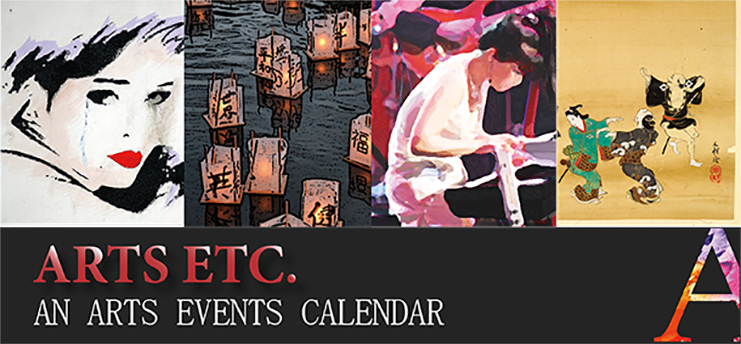The image is a visually captivating cover, possibly for a calendar or an advertisement, featuring an array of Japanese art styles and distinct elements. In the upper left-hand corner, there's a minimalist drawing of a woman with red lips and a completely white face, accentuated by sketched black hair. Adjacent to this, floating in water, are several traditional Japanese paper lanterns with candles inside. To the right, a lineless painting depicts a young woman with black hair dressed in white, seemingly engrossed in weaving or working on a craft. Further to the right, a classic Japanese painting showcases three mythological characters, each dressed in distinct colors—green, brown, and black—with the top-right figure resembling a bird. Below these elements, a sleek black banner features the text "ARTS ETC" in bold red uppercase letters, followed by "an ARTS EVENTS CALENDAR" in white uppercase letters. In the bottom right corner, the design is completed with a large, colorful stylized letter "A," formed by various art paint patterns.